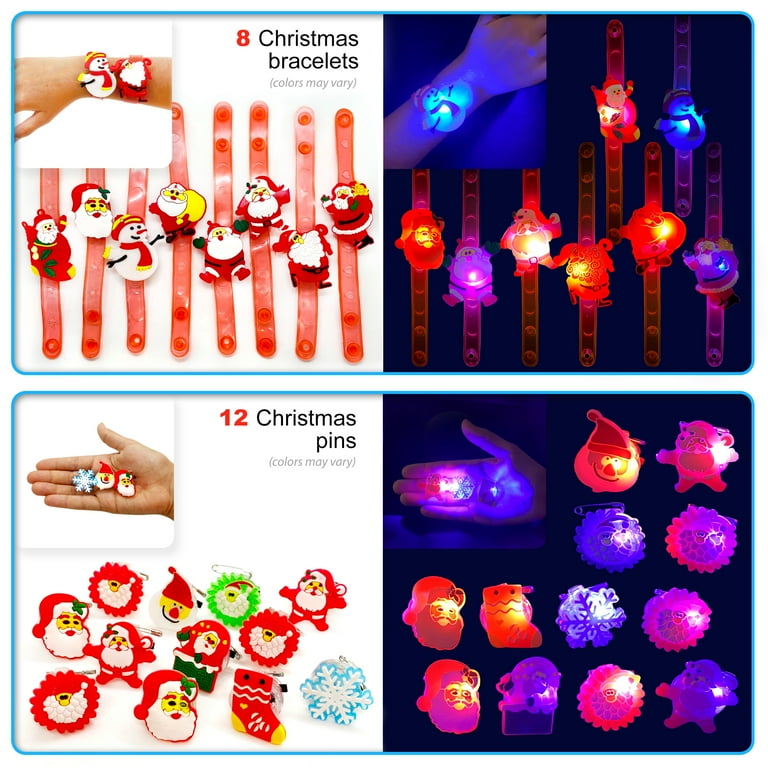This advertisement-style photo features a festive display of Christmas accessories designed to light up your holiday season. The top half of the image, framed with a light blue border, is dedicated to showcasing "8 Christmas bracelets." These bracelets come in various colors such as red, purple, and blue, each adorned with cheerful characters like Santa Claus in different poses, and a blue snowman. A close-up image illustrates two of these bracelets worn on a wrist, highlighting their vibrant, winter-themed designs. To the right, the bracelets are depicted glowing in the dark, illuminated in shades of red, pink, purple, and blue.

The bottom half mimics the top layout but focuses on "12 Christmas pins." These lapel-style pins feature a variety of holiday characters and motifs, including snowflakes, stockings, Santas, and snowmen. An image shows a hand displaying three of the pins, emphasizing their detailed designs. Beside it, the same pins are shown lit up in the dark, radiating a festive glow in colors of red, pink, purple, and blueish tones. This comprehensive advertisement captures both the intricate details and the luminous beauty of these holiday accessories.